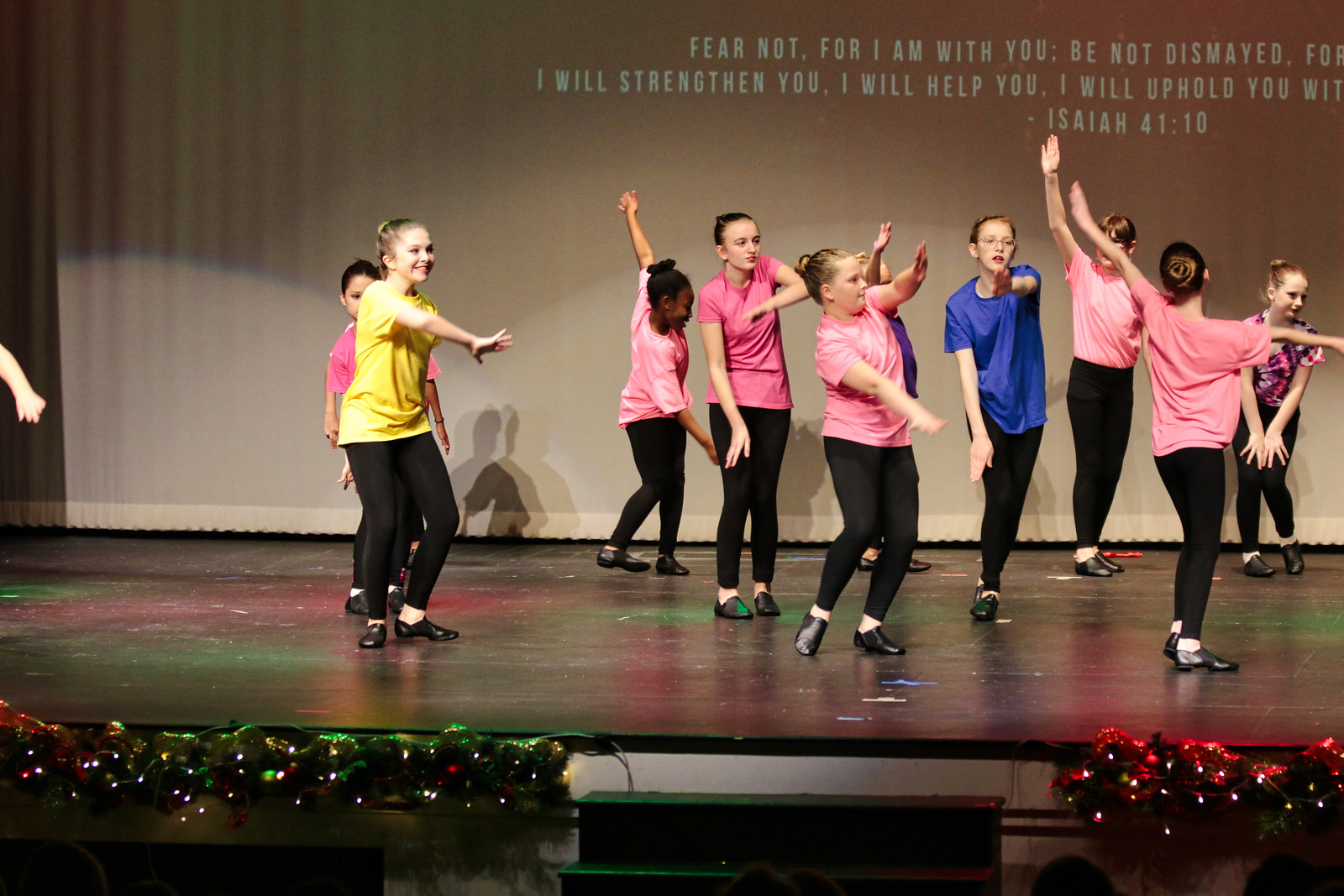This photograph, taken indoors on a rectangular stage, captures a group of young girls aged between 12 and 14 years old, dancing in a church setting adorned with Christmas decorations. The stage features green steps at the center leading up to it and is festooned with green garlands illuminated by Christmas lights. The girls, dressed in black tight pants and t-shirts in colors of pink, blue, yellow, and one in a tie-dye design, are in the midst of their dance routine, each moving with individualized, somewhat unchoreographed expressions. They are all wearing black dancing shoes and their movements include extended arms as if in a windmill pose. Behind them, a light tan curtain serves as the backdrop, onto which a biblical verse from Isaiah 41:10 is partially projected, reading, "Fear not, for I am with you; be not dismayed, for I will strengthen you, I will help you, I will uphold you…" The engaging performance and festive decorations highlight the vibrant atmosphere of the scene.